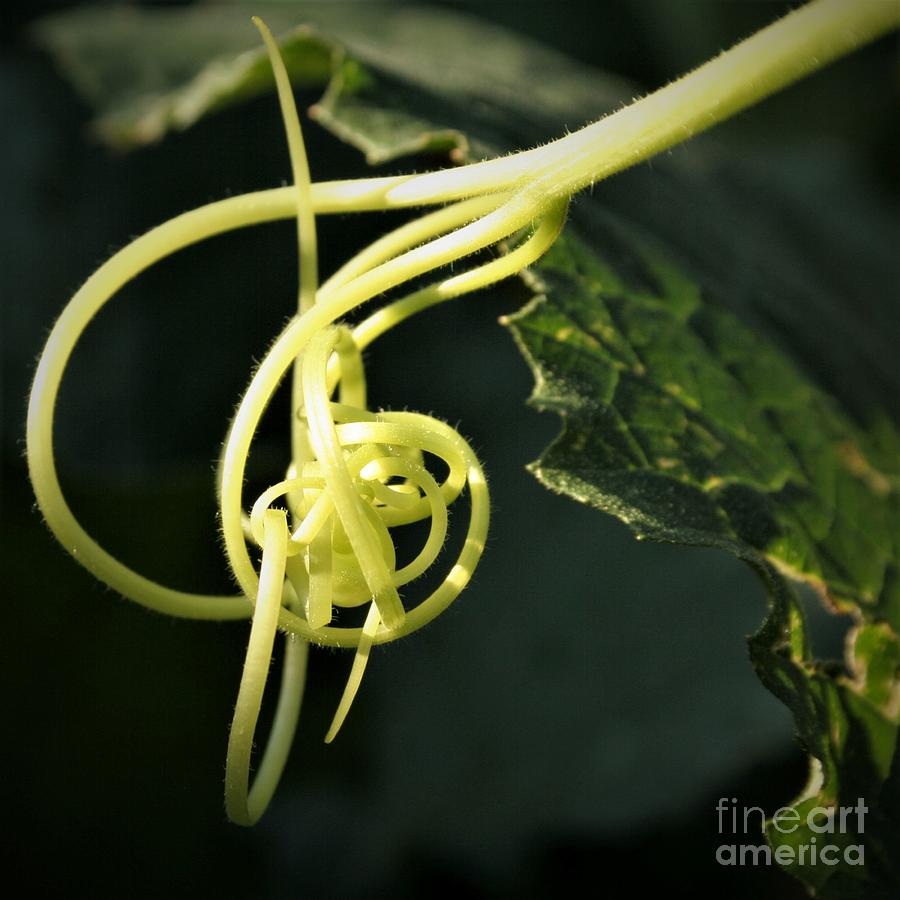In this highly detailed and close-up color photograph, we observe a fascinating part of a plant. Dominated by a bright yellow-green curly stem that loops and tangles intricately resembling knotted yarn or spaghetti, the image showcases nature's intricate designs. The fine details are so sharp that we can see tiny hair-like structures along the edge of the stem. The background provides a contrasting dark green, featuring a blurred yet recognizable green leaf with visible veins and jagged edges. The lighting masterfully highlights the curly stem, drawing attention to its complex structure. A subtle watermark reading "Fine Art America" is seen in white in the lower right corner of the image.